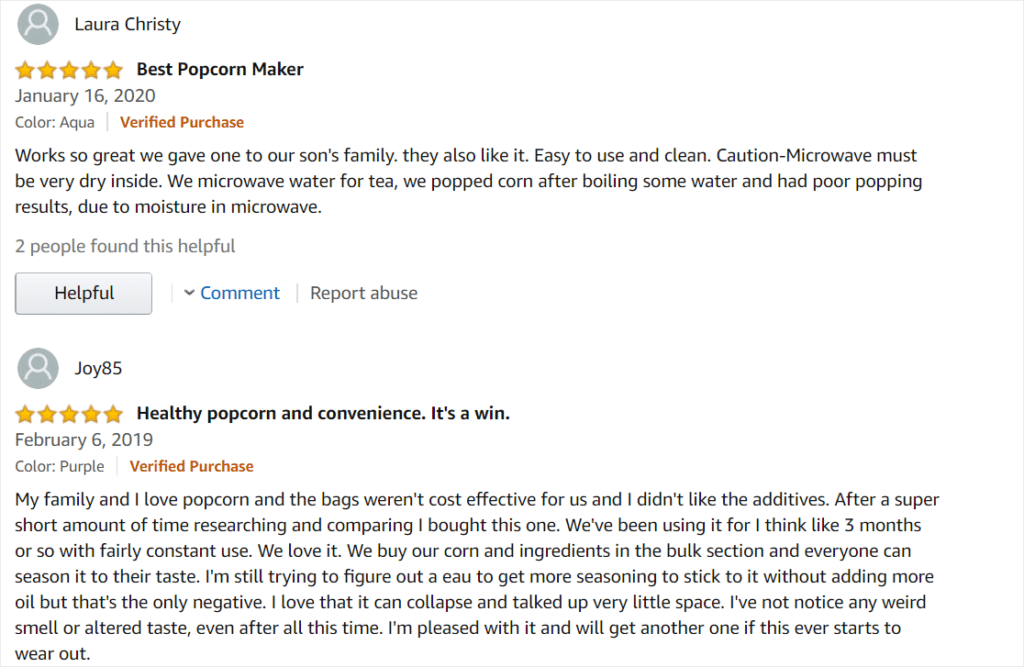This is a screenshot from my website, resembling the familiar format of an Amazon review page. In the top left corner, there's an icon featuring a silhouette of a head and shoulders in grey beside the name Laura Christie. Laura has given a five-star review for a product labeled as the "Best Popcorn Maker," dated January 16, 2020. The review details a verified purchase of the product in the Aqua color. It praises the popcorn maker for its efficacy and ease of use, noting that they even gifted another one to their son's family, who also find it convenient. However, Laura advises ensuring the microwave is thoroughly dry before use, as residual moisture interfered with their popcorn preparation.

Below this, there's a secondary review by Joy85, also rated at five stars, titled "Healthy popcorn and convenience. It's a win," dated February 6, 2019, for the purple color variant and also a verified purchase. Joy85 explains how their family opted for this popcorn maker to avoid the cost and undesirable additives of pre-packaged popcorn. After using it consistently for approximately three months, they express satisfaction with its performance, noting its space-saving design due to collapsibility and lack of residual smells or altered tastes even after extensive use. Joy85 mentions a minor drawback – difficulty getting seasoning to stick without adding more oil – but remains pleased overall and considers repurchasing if necessary.

Both reviews feature interactive elements such as a grey "Helpful" button with an indicator showing two people found Laura's review helpful, a "Comment" button with a small downward arrow in blue, and a "Report abuse" option.